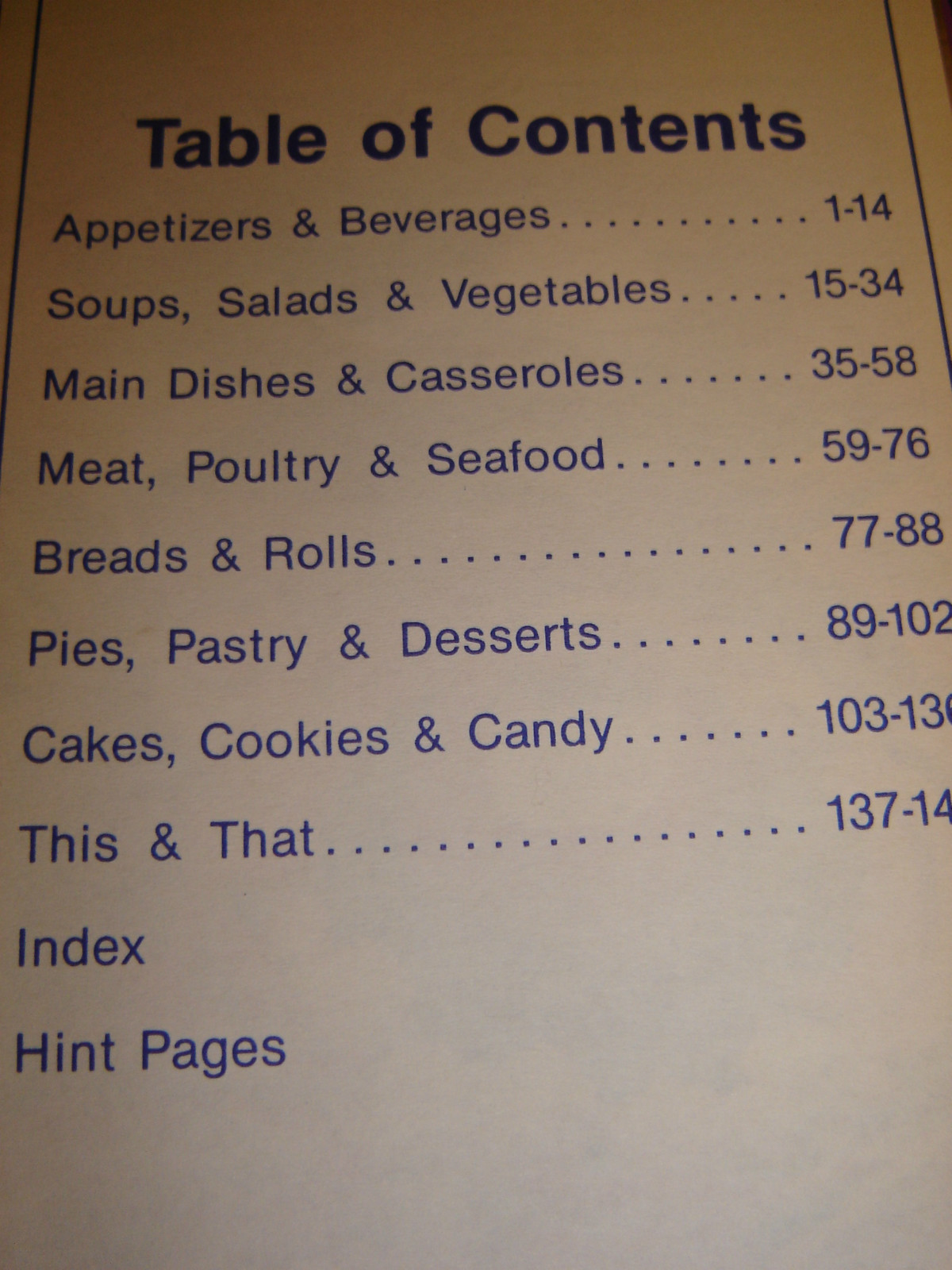A detailed and structured caption:

"A detailed photograph capturing the Table of Contents page of a cookbook. The page, set against a beige background, lists the contents in elegant blue font. It begins with 'Appetizers and Beverages' spanning pages 1 to 14, followed by 'Soups, Salads, and Vegetables' covering pages 15 to 34. Next, 'Main Dishes and Casseroles' are featured on pages 35 to 58. The section for 'Meat, Poultry, and Seafood' runs from pages 59 to 76. Following this, 'Breads and Rolls' occupy pages 77 to 88, and 'Pies, Pastries, and Desserts' are detailed from pages 89 to 102. The next section, 'Cakes, Cookies, and Candy,' extends from page 103 to page 136. The last category visible is 'This and That,' starting from page 137, although the final page number is cut off in the image. Additionally, the table includes lines for 'Index' and 'Hint Pages,' completing the comprehensive organization of the culinary contents within the book."